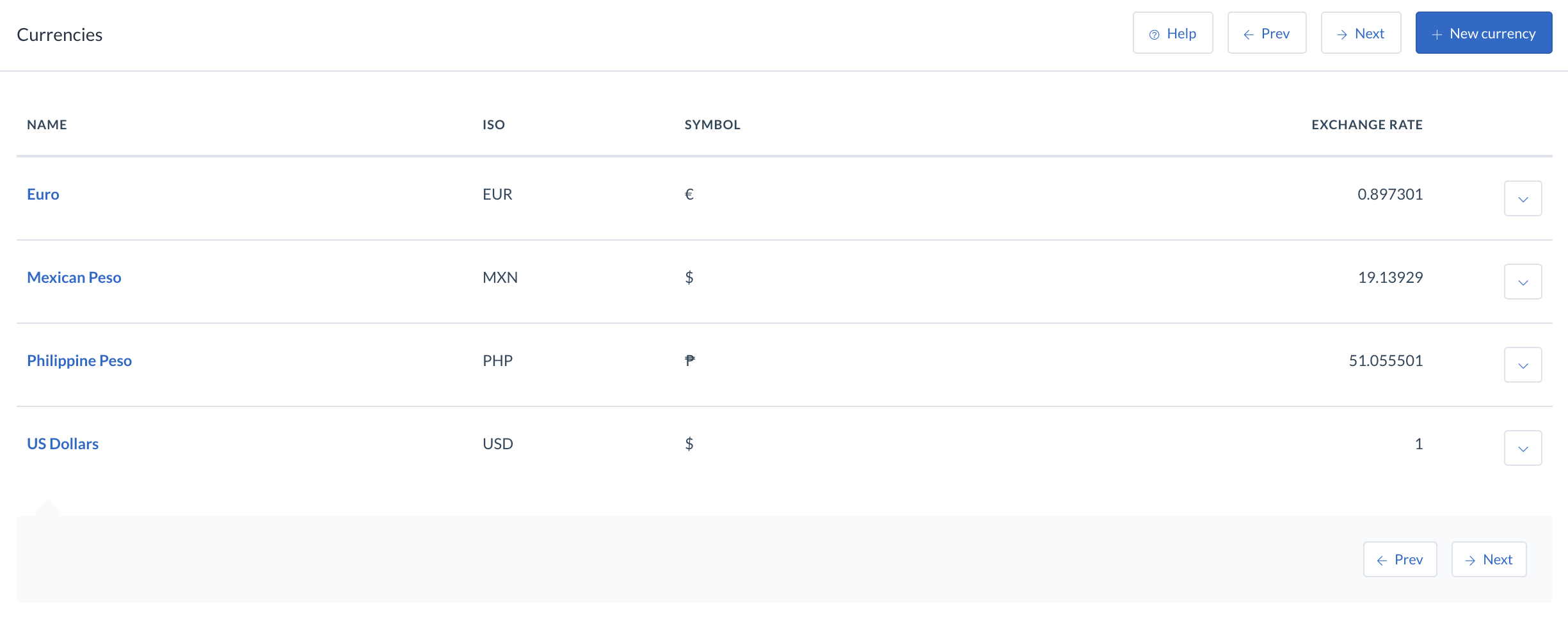This image displays a table listing various currency exchange rates, likely sourced from a website, although the site's name is not visible or may be cut off. At the top left, there is a clear header labeled "Currencies" in black and white text. On the top right, options for "Help," "Previous," "Next," or "New Currency" are available.

Directly beneath this top section, the table columns are labeled as follows: "Name," "ISO," "Symbol," and "Exchange Rate." The rows of the table outline specific currencies along with their respective details:

1. The first row lists the Euro:
   - Name: Euro
   - ISO: EUR
   - Symbol: €
   - Exchange Rate: 0.897301

2. The second row represents the Mexican Peso:
   - Name: Mexican Peso
   - ISO: MXN
   - Symbol: $
   - Exchange Rate: 19.13929

3. The third row details the Philippine Peso:
   - Name: Philippine Peso
   - ISO: PHP
   - Symbol: ₱
   - Exchange Rate: 51.055501

4. The fourth and final row lists the U.S. Dollar:
   - Name: U.S. Dollar
   - ISO: USD
   - Symbol: $
   - Exchange Rate: 1

Overall, this image precisely captures the current exchange rates of these currencies against a base currency, likely providing essential information for financial analysis or international transactions.